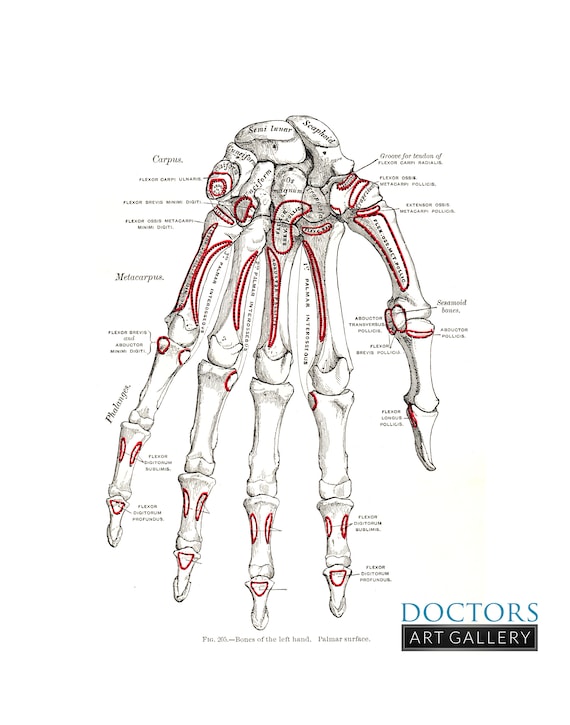The image depicts an educational anatomy illustration of the human hand, specifically focusing on the bones and their associated structures. Centered on a white background is a detailed drawing of the left hand's palmar surface, showcasing the skeletal framework in a large, zoomed-in view. The bones, rendered in white, are meticulously labeled with minute, red-highlighted annotations indicating various parts such as the wrist bones, carpal bones, and phalanges, among others. Names of specific bones like the semilunar, scaphoid, cruciform, and trapezoid are visible, although much of the smaller text remains difficult to read. Distinctive red lines point to particular areas, denoting the importance of muscles and other anatomical features, including terms like carpus, flexor carpi ulnaris, flexor brevis, and flexor digitorum profundus. At the bottom right corner, a black and gold banner, reading "DOCTORS ART GALLERY" in white capitals, underlines the image. Below this banner, a caption in blue capitals states "Bones of the Left Hand, Palmar Surface."